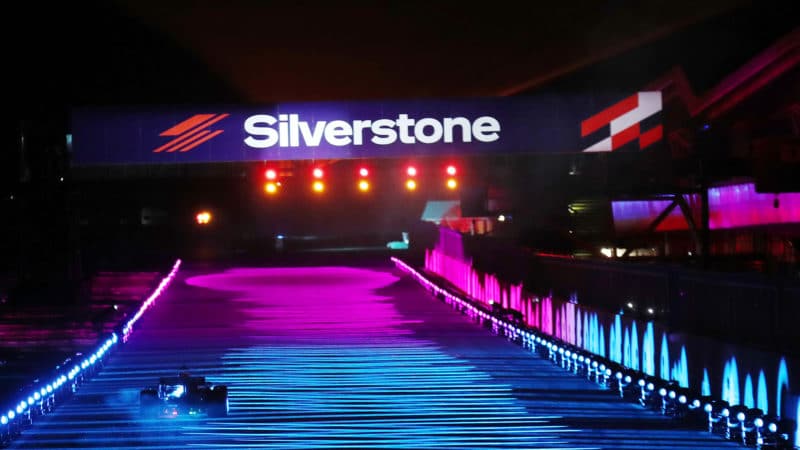The photograph depicts a nighttime scene at a racetrack, viewed straight ahead onto the paved surface. The foreground of the track appears very dark navy blue due to the lighting, while the background is illuminated in a vivid hot pink or magenta. A small race car, mostly indistinguishable except for the visibility of its wheels, is positioned on the track.

Above the track hangs a blue, rectangular banner with the word "Silverstone" boldly written in white letters. Flanking the word on either side are red geometric logos. The lighting and overall color palette of the image ranges from red to purple to blue, creating a striking contrast against the dark surroundings. In addition to these primary elements, the image features some colorful lights and possibly fountains, enhancing the vibrant atmosphere of the scene. Despite the overall darkness, the image is clear and well-defined.